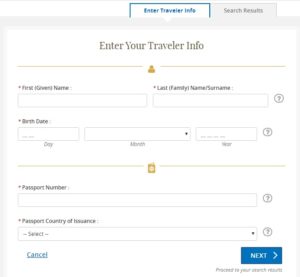The vertical image depicts a detailed user interface for entering traveler information on a website. At the top of the screen, there are various tabs, with one outlined in turquoise. This highlighted tab has bold turquoise text in the center reading "Enter Traveler Info." To the right, another tab labeled "Search Results" is shown in gray font.

In the center of the screen, large gray text prompts users to "Enter Your Traveler Info." Below this prompt is a horizontal line with an icon in the center, though the icon is difficult to discern.

The form fields are laid out on a crisp white background. The first field is labeled "First Name, First Guest Name" and features a horizontally rectangular input box marked with a red asterisk, indicating it is required. To the right of this, the label reads "Last Family Name, Surname."

Below, there is a section for birth date information with three input boxes labeled "Day," "Month," and "Year" respectively. Following this section, there's another horizontal line in light green with an indistinct yellow or gold icon at its center.

The subsequent field is labeled "Passport Number" in what appears to be bold black font, accompanied by a horizontal input box. Further down, the "Passport Country of Insurance" field includes a pull-down menu to select the country. The interface also contains two buttons at the bottom: a blue, underlined "Cancel" button on the left and a "Next" button on the right with a blue background and white text.